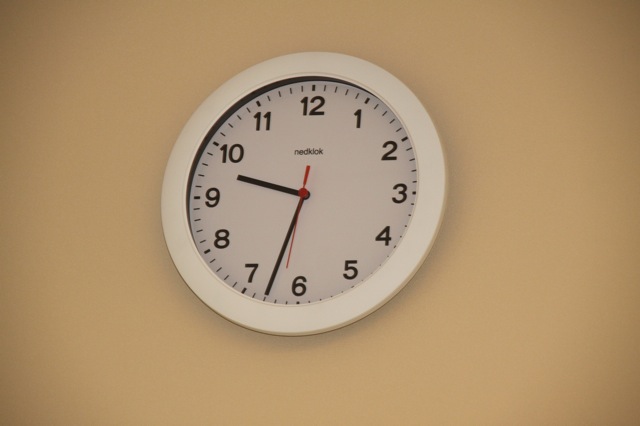The photograph depicts a white wall clock with bold black numerals ranging from 1 to 12, hanging on a tan-colored wall. The clock features a round white frame and a matching white center. Its minute hand and hour hand are black, while the second hand stands out in red. Minute markers are represented with small lines between the numbers. The clock displays the time as 9:33 and 31 seconds. Just below the number 12, the brand name, which appears to be spelled "N-E-D-K-L-O-K," is subtly printed. The clear, color photograph captures the clock as the main focal point, possibly for a sale listing.